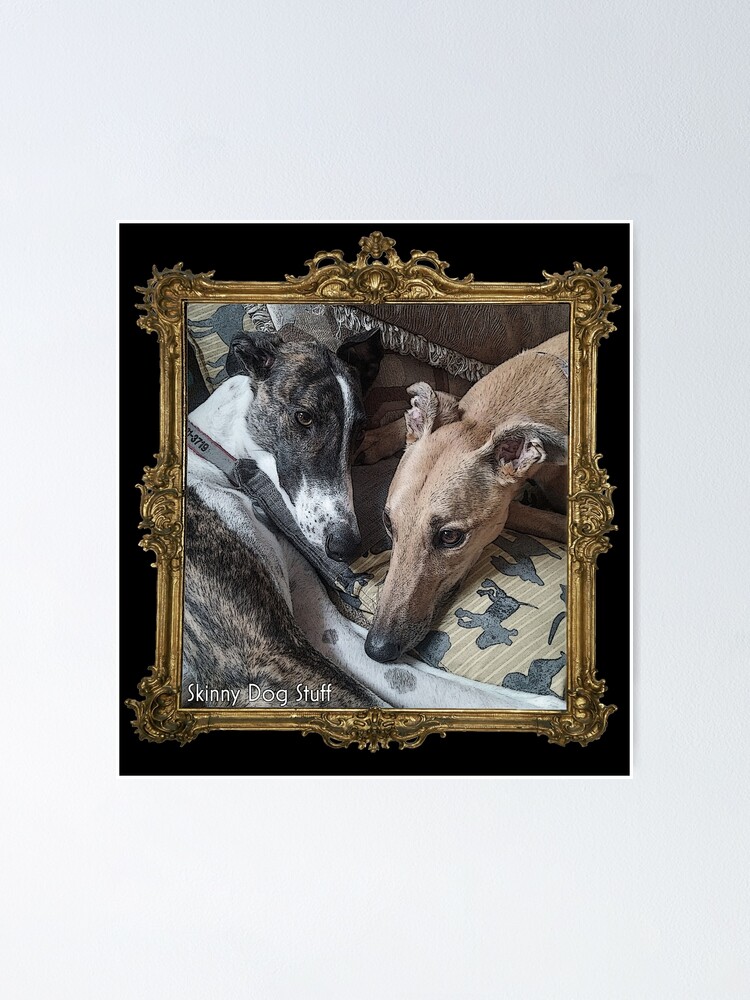This image features a detailed painting of two greyhounds resting on decorated bedding. The painting, framed in an intricate gold frame with elaborate designs, displays a grey and white greyhound facing right and a light blondish greyhound facing left, with its nose gently resting on the other greyhound's limb. The scene is set within a black background, forming an inner square, which is further enclosed within a light blue rectangular border. The text "Skinny Dog Stuff" is prominently featured in white in the lower left-hand corner of the painting.